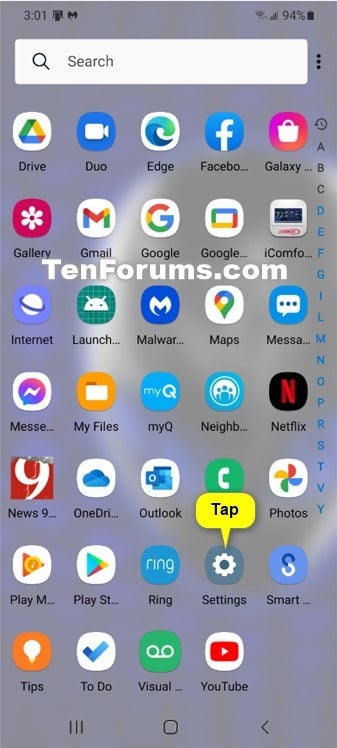The screenshot shows an iPhone with a timestamp of 3:01 PM and a battery level at 94%. The home screen is densely populated with various apps including Galaxy Duo, Google Drive, Microsoft Edge, Facebook, and Netflix, among others, filling the entire page. A prominent yellow pop-up appears, instructing the user to "tap under settings". The image is watermarked with "tenforms.com", suggesting it might be part of a review highlighting the new home screen layout at the time of the phone's release. The overall design and app icons indicate that the screenshot is likely from an iPhone released around ten years ago.